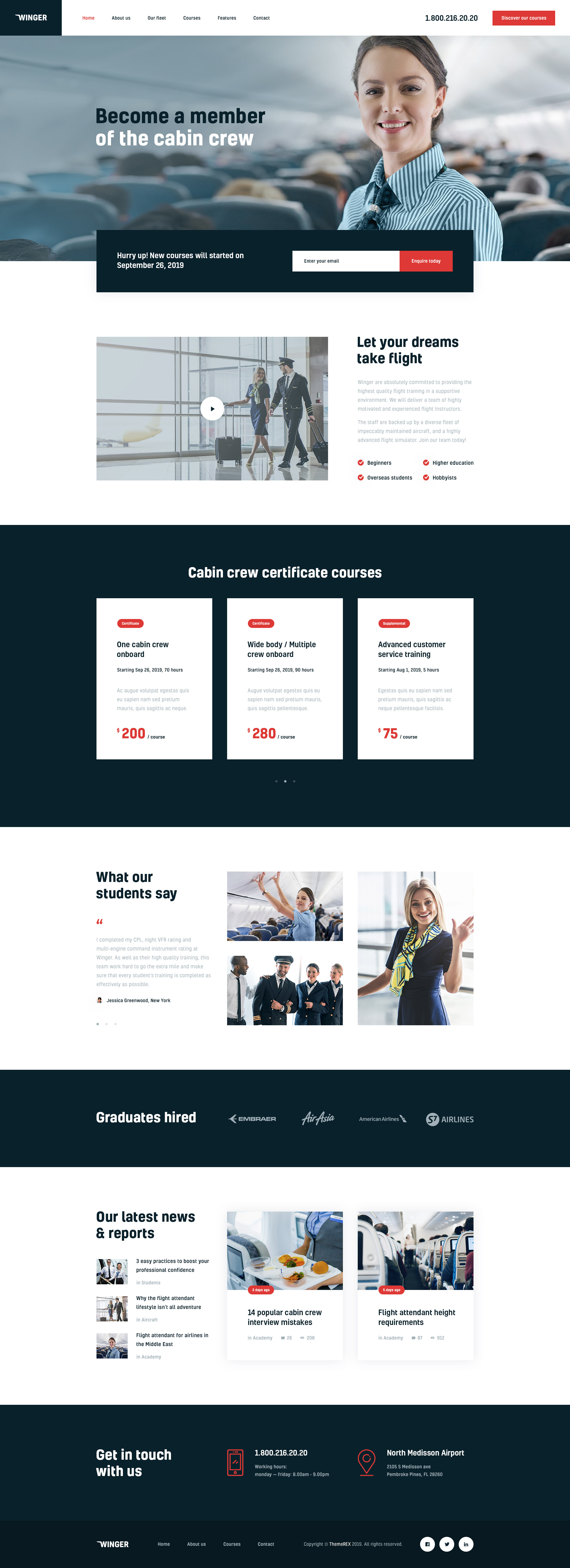**Detailed Caption for the Screenshot from a Smartphone Display**

The image is a detailed screenshot from a typical smartphone interface. At the very top, there is a white border featuring a search bar and a small black rectangular icon with white text inside. The rest of the header is predominantly white, transitioning from left to right. Immediately following the black box, there is a segment with six words in black, with the first word post-black box rendered in a reddish hue. Continuing to the far right, additional black text appears followed by another black rectangular box housing white text.

Below this header section, there is a prominent rectangular photograph. The photo depicts a smiling woman with a fair complexion, wearing a blue striped shirt paired with a tie, her hair neatly tied back. The photograph's context suggests she is potentially a flight attendant, as indicated by the text "Become a member of the cabin crew" in white lettering on a black background on the left-hand side of the photo. Behind her, the airplane fuselage, ceiling, and partial views of passengers' heads and seats are visible, enhancing the airline setting.

Directly beneath this image, there is a small black rectangular box with white text situated on the left, and another smaller rectangular box partially cut off on the right, featuring a red box with white text in the center. Below this, a circular icon with a black dot in the middle appears alongside another image. This second image shows the same woman, now in an airport, wheeling a black suitcase and conversing with a man in a suit and cap, presumably an airline colleague. Text to the right in black letters reads, "Let your dreams take flight."

Further down, four bullet points in black text are listed, followed by another black rectangular box with white letters proclaiming "Cabin Crew Certification Courses." This section showcases three distinct rectangular boxes at the bottom, each marked with an oval red tab on the left corner, black text beneath, and a light gray paragraph. The pricing details are visible: $200, $280, and $75 respectively.

Towards the middle of the screenshot, a black and white section houses the heading "What Our Students Say", followed by a gray paragraph and a black quote. Three smaller accompanying images display a flight attendant assisting with luggage, a diverse group of crew members including a captain and two women, and a woman waving with her hair down.

Near the bottom, the section highlights "Graduates Hired" with a black rectangular background and four slogans. Three more images below promote "Our Latest News and Reports," each accompanied by captions in black text. Another set of two images, with a red button in the bottom left corner, showcases airplane seats and aisles.

The screenshot concludes with a large black rectangular box stating "Get in Touch with Us" in lighter lettering. Adjacent to this, a red logo on a black background with white text appears, along with another red logo featuring similar white text. Small, barely legible icons span across the bottom, ending with three circles each containing a dot in the center.